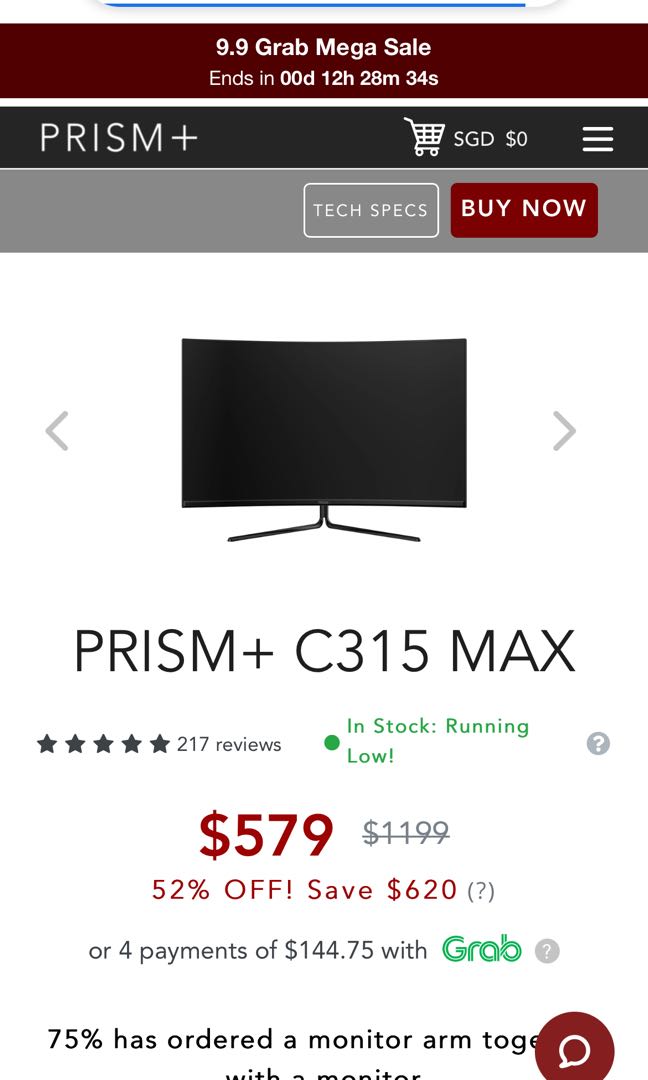**Descriptive Caption:**

The image is a colorful snippet from a website showcasing a special offer. At the top, a thin blue bar spans the width of the page. Below it lies a brown rectangle with white text announcing a "9.9 Grab Mega Sale" that ends in "00 days, 12 hours, 28 minutes, 34 seconds."

Directly underneath, a dark grey rectangle bears the text "Prism Plus" in white, alongside icons for a cart, indicating SGD50, and a hamburger menu. Below this, a lighter grey rectangle hosts two buttons: a "Text Specs" button outlined in white and labeled in white text, and a "Buy Now" button in dark burgundy with white writing.

The main section has a white background featuring a central image of a black computer monitor, which is turned off and has two black legs. Adjacent to the monitor are forward and backward navigation icons. The model, "Prism Plus 315 Max," is displayed along with a five-star rating and 217 reviews. A note indicates that the item is in stock but running low. The price is prominently shown as $579, reduced from $1199, marking a 52% discount. Customers can save $620 or choose an installment plan of four payments of $144.75 with 'grab,' highlighted in green. 

Additional information mentions that 75% of customers have ordered a monitor arm with their purchase. In the lower right corner, partly obscured text appears under a round brown icon with a white question bubble. Some of the bottom text is partially cut off and unreadable.